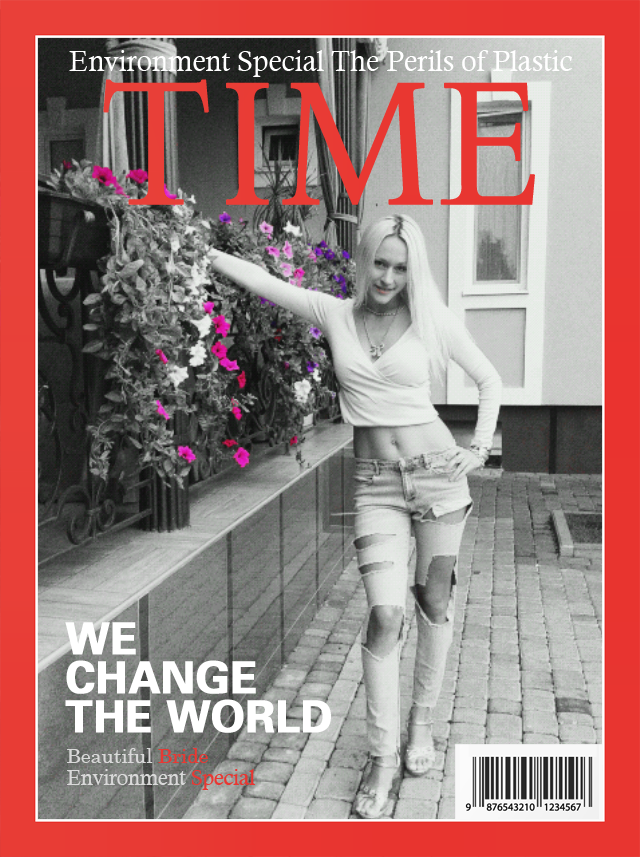The cover of the Time magazine features its iconic all-red border and bold, red "TIME" title. Dominating the black-and-white image is a confident, blonde-haired woman in a revealing white blouse that shows her midriff, along with ripped jeans that expose her thighs, and she's wearing sandals. Her left hand rests on her hip as she leans against what appears to be a couple of pillars to her right, decorated with vibrant flowers in shades of magenta, pink, purple, and red, adding a touch of color to the monochromatic photograph. The cover also includes various texts: at the very top, it reads "Environment Special: The Perils of Plastic," while towards the bottom left, it states, "We Changed the World, Beautiful Bride." Additionally, a barcode is visible at the bottom right corner of the cover.